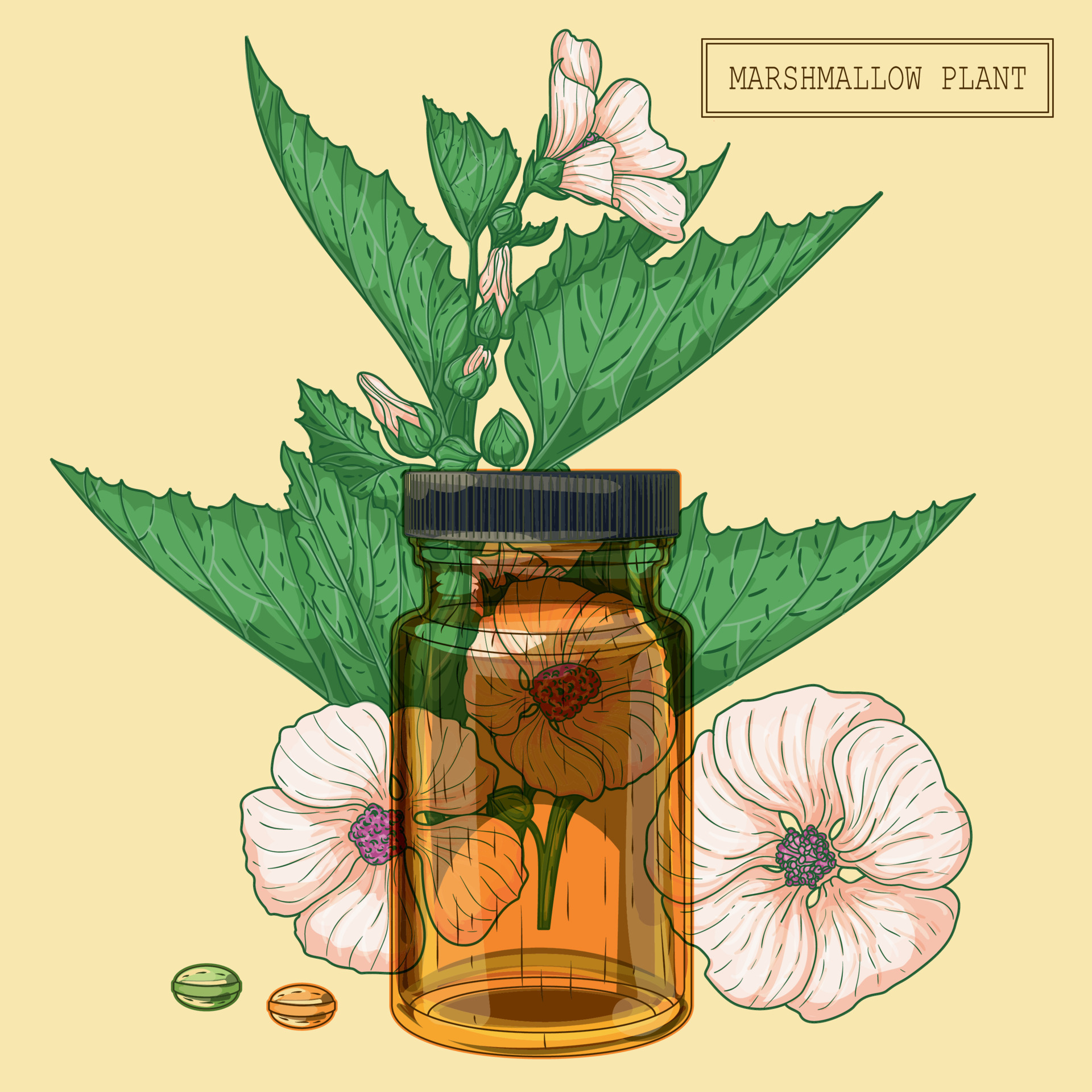This image is a digital painting of a marshmallow plant, set against a beige background. In the upper right corner, within a black-bordered box, the black text reads "marshmallow plant." The plant, centered in the image, features vibrant green leaves with sawtooth edges and large flowers. The flowers have white petals with purplish and green centers, and some are fully bloomed while others are still budding.

In the foreground, a transparent, amber-tinted cylindrical jar with a black lid partially obscures the lower part of the plant. Through the jar, you can see three prominent flowers facing outward, their centers fully exposed. On the surface at the bottom left are two objects resembling pills or seedlings, one green and one brown. The detailed portrayal of the plant and the jar against the tan background creates a striking and detailed composition.